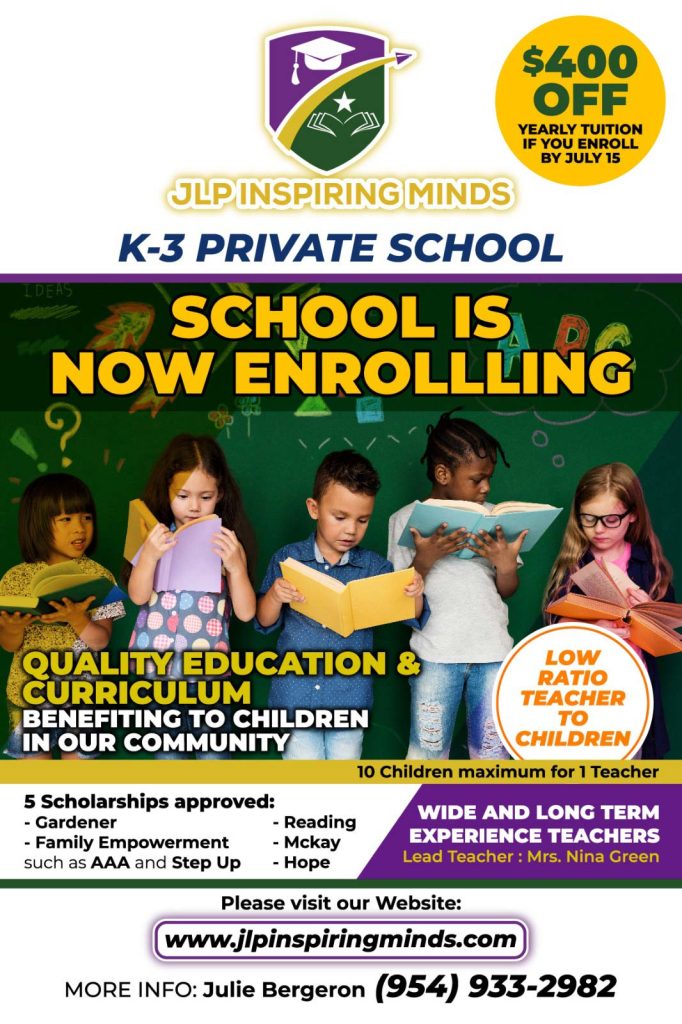This detailed ad for JLP Inspiring Minds, a K-3 private school, features a prominent shield shape at the top, divided by a yellow arc. The upper section is purple, containing a white graduation cap, while the lower green section holds the white outline of a book with a star above it. At the apex of the arc sits a small purple paper airplane. 

To the right of the shield is a yellow circle with text offering "$400 off yearly tuition if enrolled by July 15th." Below the shield and yellow circle, bold text reads "JLP Inspiring Minds," followed by "K-2-3 Private School." 

The main image shows young children engrossed in reading, overlaid with the text "School is now enrolling" at the top. In the bottom left corner, text highlights the school's commitment: "Quality education and curriculum benefiting children in our community." The bottom right corner of the image features a white circle stating "Low ratio: teacher to children."

At the very bottom, a yellow bar emphasizes "10 children maximum per teacher." Below the bar is additional information about scholarships, teacher experience, and contact details, ensuring that prospective parents have all the necessary information to consider enrolling their children.